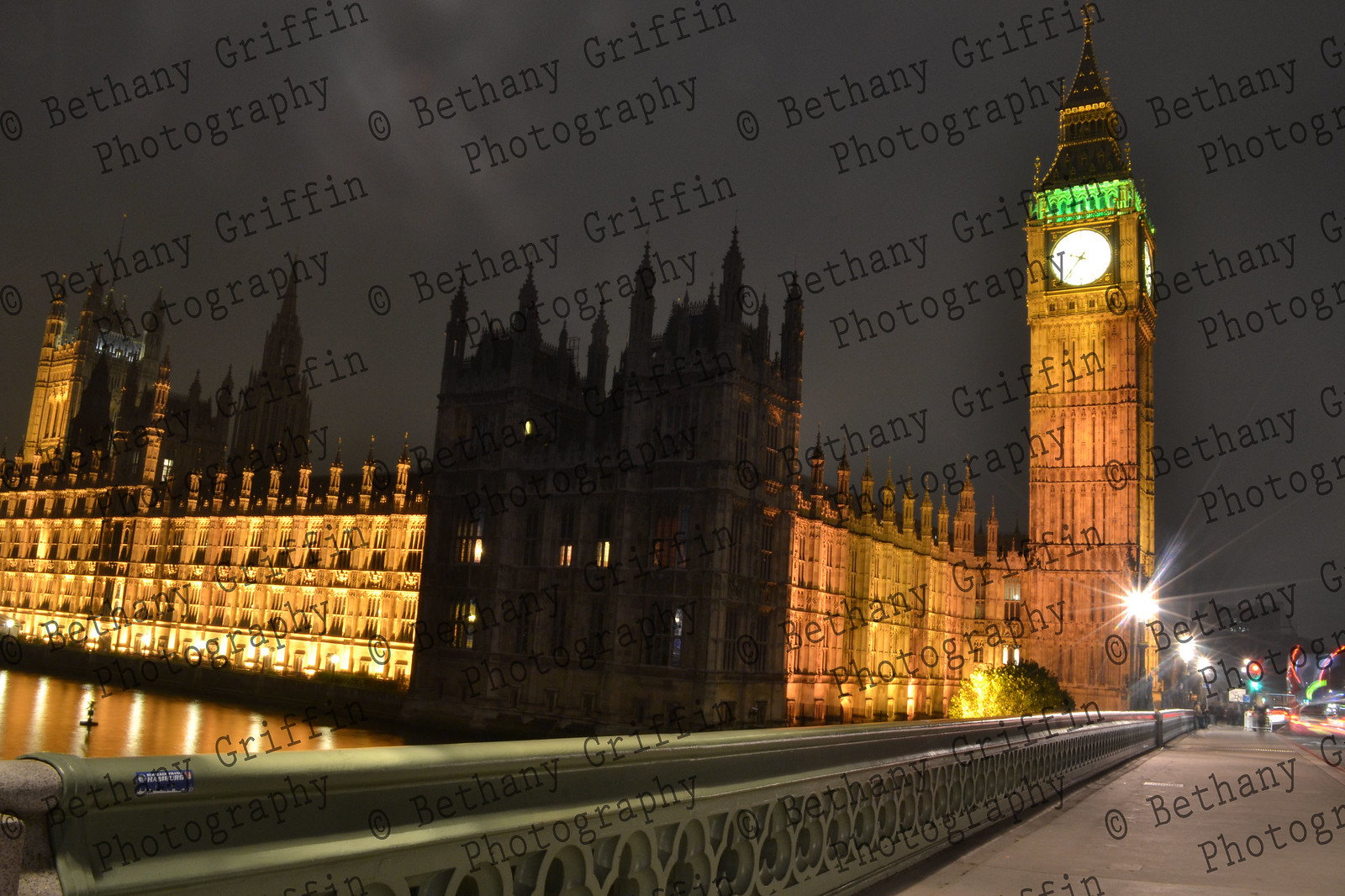In this photograph taken by Bethany Griffin, we see the iconic Big Ben clock tower in London, beautifully illuminated against a pitch-black night sky. The clock face and portions of the tower are bathed in bright light, showcasing the structure's green and brown hues. The famous site is part of a larger building complex, whose left side is also lit up while the central part remains in shadow. The scene is captured from a nearby bridge, visible on the right, adding dynamic angles to the composition. Below, blurred streaks of light from passing cars on the street indicate a long exposure shot, adding an element of motion to the stillness of the grand architecture. Streetlights cast a bright, white glow, and the reflections from the lit buildings shimmer in the waterway beneath. The entire image is watermarked repeatedly with "Bethany Griffin photography" to protect her work.